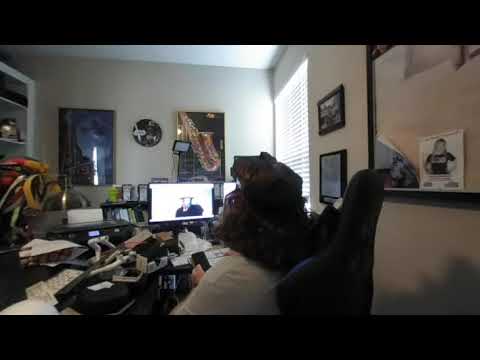This photograph depicts a woman seated at a cluttered black desk in an office-like room. Captured from behind and slightly to the side, the image doesn’t show her face but highlights her brown, shoulder-length hair and white shirt. She rests on a tall, cushioned office chair with sports car-like shoulder rests, accented by purple trim. The desk is extremely cluttered, featuring a myriad of items, possibly including guitar or backpack straps, amidst the disarray.

To her right, there is a brightly lit TV or monitor, its screen largely white, while she holds a TV remote control in her hand. The room's backdrop includes a doorway, a white wall adorned with a clock, and a black-framed poster of a saxophone. Another framed image appears to the right, along with a window fitted with white Venetian blinds. A black printer is visible to the left of the desk, adding to the busy scene. The overall clutter and the mixture of office and personal items define the photograph's atmosphere, emphasizing the woman's absorbed engagement with the TV or monitor.